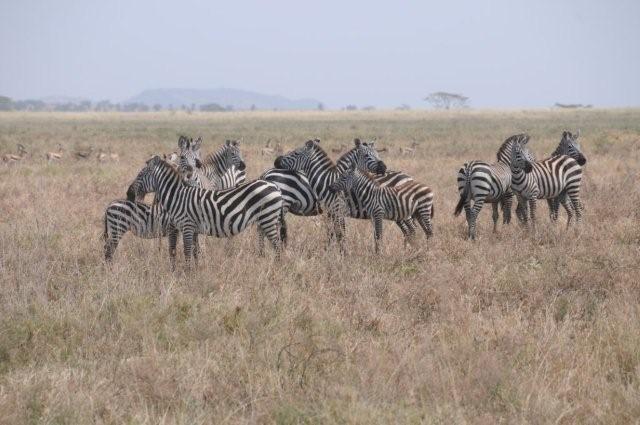In this slightly faded daytime photograph, a herd of zebras stands in a drought-affected savanna. The flat landscape, dominated by tall, dry, brown grass with sparse patches of green, stretches to the horizon under a hazy blue sky. There appear to be around seven to nine zebras, all adults, oriented in various directions; some are grazing with heads down, others are vigilant, looking out across the field. Behind them in the background, a faint line of antelopes can be seen crossing, accompanied by a distant outline of trees and a subtle mound to the left. This vivid depiction captures the essence of the wild African prairie.